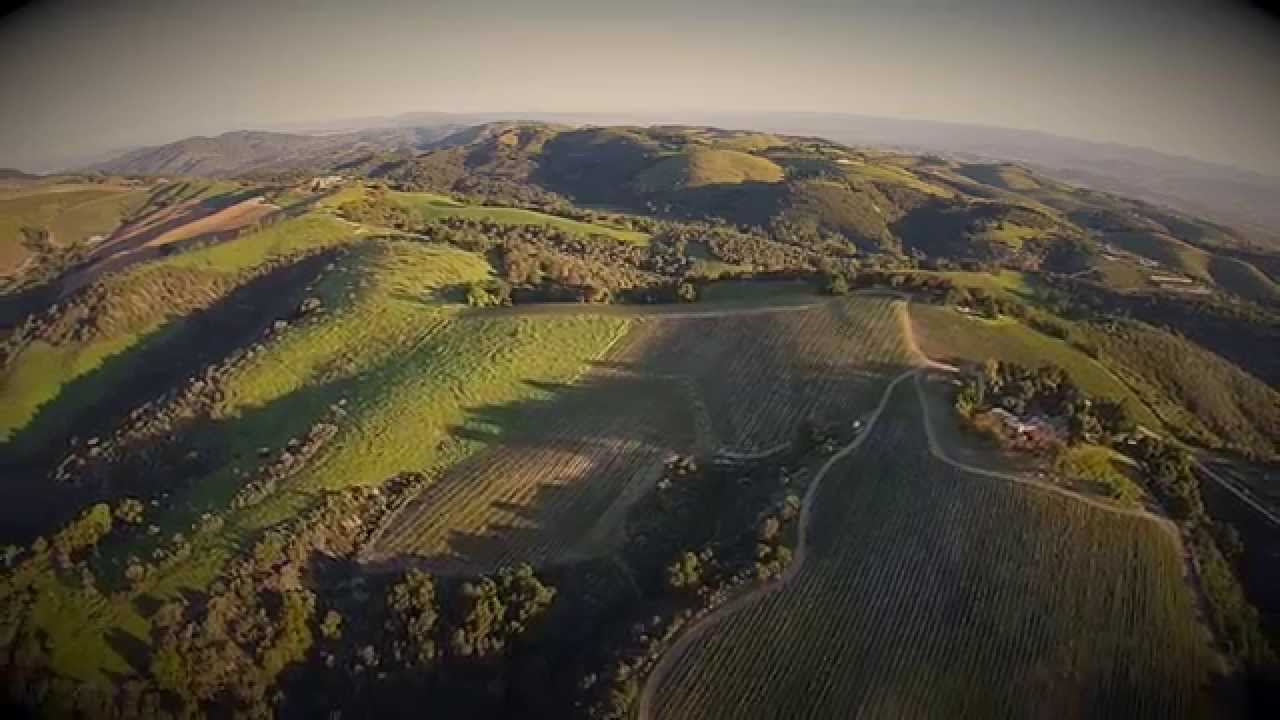This overhead, bird's-eye view captures a sprawling, lush green mountain interspersed with agricultural fields and crisscrossed by winding paths and roads. The photo is taken from a significant altitude, possibly by a drone or airplane, offering a detailed panorama that makes the terrain appear to curve slightly, suggesting the use of a fisheye lens. The image has a vignette effect, darkening towards its rounded corners. The sky above the landscape appears overcast and hazy, either due to the natural weather conditions or as a result of post-editing, lending a moody and atmospheric quality to the scene.